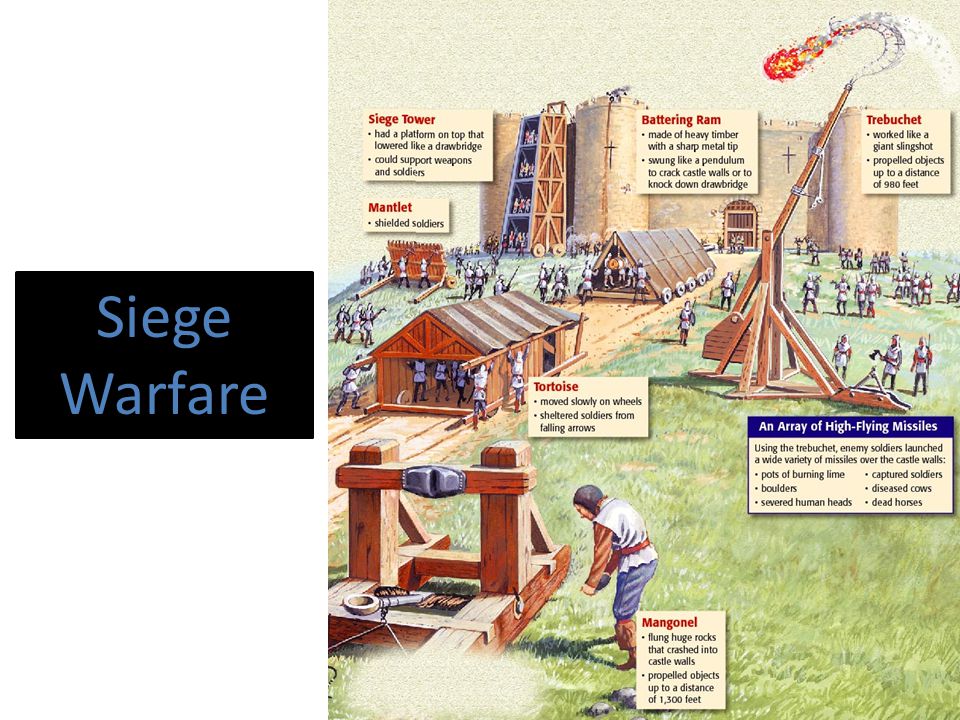The infographic, entitled "Siege Warfare," features a detailed illustration highlighted by a prominent black rectangle on the left, bearing the title in light blue text. Dominating the right side is a rich, colored-pencil drawing that vividly depicts a medieval siege scenario. The central focus is a tan stone castle marked with two crosses and a brown door, positioned in the background. 

A dirt path, flanked by two tents that serve as outposts for soldiers, leads up to the castle. Along this path is a tapestry of siege weaponry: a towering siege tower under construction on the castle's left, a battering ram positioned on the road, and a tortoise—a wheeled, protective structure—trailing behind it. A mangonel catapult is stationed in the foreground, operated by a man loading a rock.

Additionally, there's a trebuchet launching a flaming projectile at the castle, situated near another text box describing a variety of high-flying missiles. Each of these mechanical contraptions is accompanied by explanatory text boxes, detailing their names, functions, and usage. The grass in the scene is colored a light green, enhancing the historic and tactical atmosphere of the artwork.